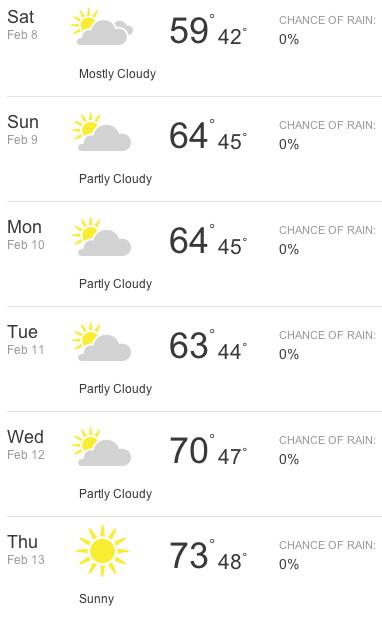The image depicts a weather forecast for an unspecified location, covering the period from Saturday, February 8th, to Thursday, February 13th. The forecast is organized in a vertical stack of rectangular boxes, each representing a day. Here's a detailed breakdown of the weather for each day:

- **Saturday, February 8th:** The forecast shows a yellow sun partially obscured by gray clouds, indicating it will be mostly cloudy. The high temperature is 59°F, while the low temperature is 42°F. The chance of rain is 0%.
  
- **Sunday, February 9th:** The weather remains partly cloudy with the same icon of a sun partially obscured by clouds. The high temperature increases to 64°F, and the low to 45°F. The chance of rain remains at 0%.
  
- **Monday, February 10th:** Similar to the previous day, it is partly cloudy with a high of 64°F and a low of 45°F. The chance of rain continues to be 0%.
  
- **Tuesday, February 11th:** The weather forecast is partly cloudy once again with a high of 63°F and a low of 44°F. The chance of rain is 0%.
  
- **Wednesday, February 12th:** Partly cloudy conditions persist, but the temperatures rise to a high of 70°F and a low of 47°F. The chance of rain remains 0%.
  
- **Thursday, February 13th:** The weather forecast predicts sunny conditions with a bright yellow sun icon. The high will be 73°F, and the low will be 48°F. There is a 0% chance of rain.

This visual representation provides a concise and clear overview of the weather for the specified period, emphasizing sunny and partly cloudy conditions with no expected rainfall. All days include both high and low temperature readings, and each day’s forecast consistently shows a 0% chance of rain.